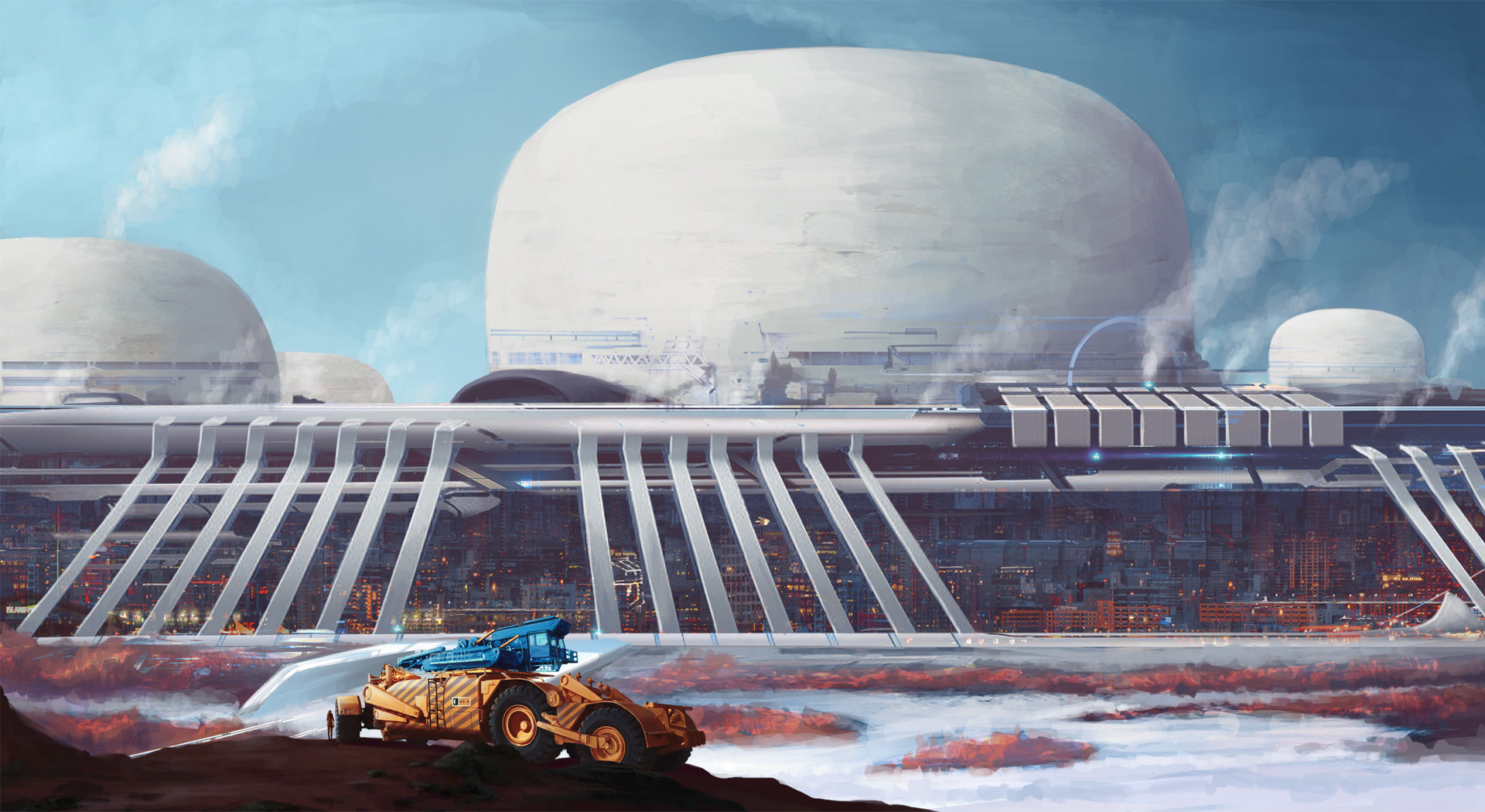The image appears to be a highly detailed, computer-generated scene evocative of a sci-fi movie setting. Dominating the background is an enormous, futuristic structure composed of four large, white, dome-shaped huts perched on a metallic, flat-roofed building. This building features numerous lights on the inside and is supported by diagonal metal beams. The setting strongly resembles a space station, reminiscent of something from Star Wars or an attraction at Disneyland like Space Mountain. There are gaps and tilted metallic bars that could be part of a fencing system. The landscape below is a reddish-orange terrain with minimal green vegetation and a mound of brown dirt on the left side. In the foreground, there's a prominent six-wheeled vehicle, yellow-orange in color with large, tractor-like tires and black stripes. Atop this vehicle is a blue apparatus, possibly a weapon or tool. The sky above is a vibrant blue with a few drifting white clouds, heightening the otherworldly atmosphere of the scene.